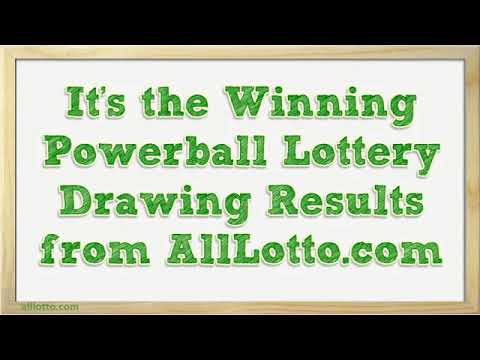The image features a clean, minimalist design with a pure white background framed by a light brown wooden border. There are strips of black letterboxing at the top and bottom of the image. In the center, the text is formatted in four lines with a medium grassy green color, giving it a subtle 3D effect with striations running from the upper right to the lower left, adding some texture to the letters. The text reads, in large, capitalized letters: "It's the winning," on the first line, followed by "Powerball Lottery" on the second line, "Drawing Results" on the third line, and "from AllLotto.com" on the fourth line. AllLotto.com is also capitalized for "A" and "L." The whole text is designed to pop against the white background, making it highly legible and striking.